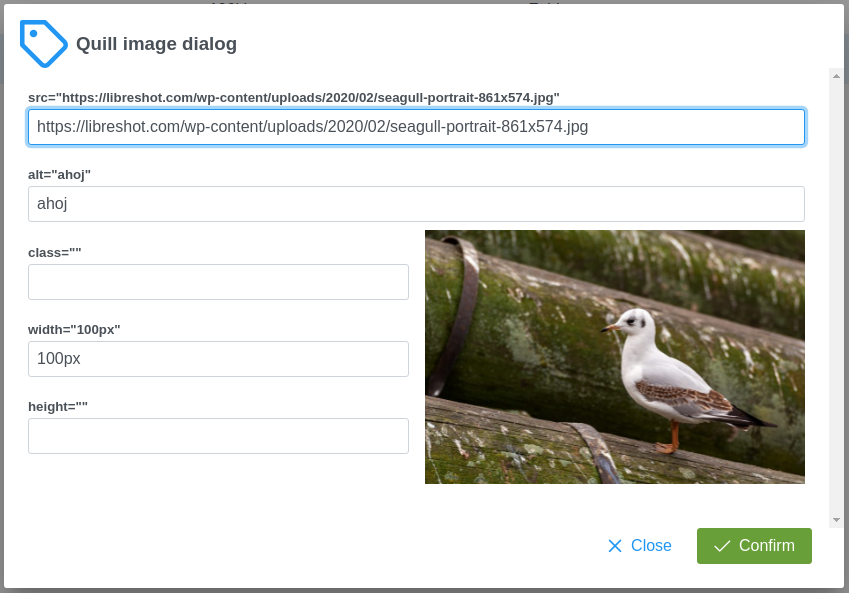The image depicts a structured webpage layout with various elements and annotations. Here's a detailed description of the visual elements as captured:

The overall design features a large rectangle with a thick gray border encompassing the entire content. At the top of this area, a small, blue tag is positioned, pointing towards the top left. The tag has a blue outline and a white center, distinguished by a blue dot in the middle, suggesting a hole for attachment.

Adjacent to this tag, towards the right, the black text reads "Quill Image Dialog." Directly below, there is a hyperlink formatted as a textual representation, which reads: `src = "https://libreshot.com/wp-content/uploads/2020/02/seagull-portrait-861-574.jpg"`.

Next, a centrally-aligned rectangular box with a blue border contains another link without the initial `src =` and quotation marks, displaying only `https://libreshot.com/wp-content/uploads/2020/02/seagull-portrait-861-574.jpg`.

Beneath this blue outlined box, non-bordered text states: `alt = "ahoj"`. Following this, another text box bordered in gray contains the word "ahoj."

Continuing downward, it reads `class = ""` followed by an empty gray-bordered box.

Midway through the page, a nearly square image of a seagull appears. The seagull, predominately white with brown edges on its wings, stands atop moss-covered logs. The logs are large and stacked, with the seagull perching on one.

To the left of this image, further descriptive text labels various dimensions and attributes:
- `width = "100px"`, accompanied by a gray-bordered box displaying "100px."
- `height = ""`, followed by another empty gray-bordered box.

Below the seagull image, two links are presented on the right. The first link, marked with an "X" and labeled "Close," is in blue. Adjacent to it, a green rectangle with a centered white checkmark reads "Confirm."

This structured layout showcases a combination of descriptive tags, links, and textual annotations related to an image of a seagull on logs.